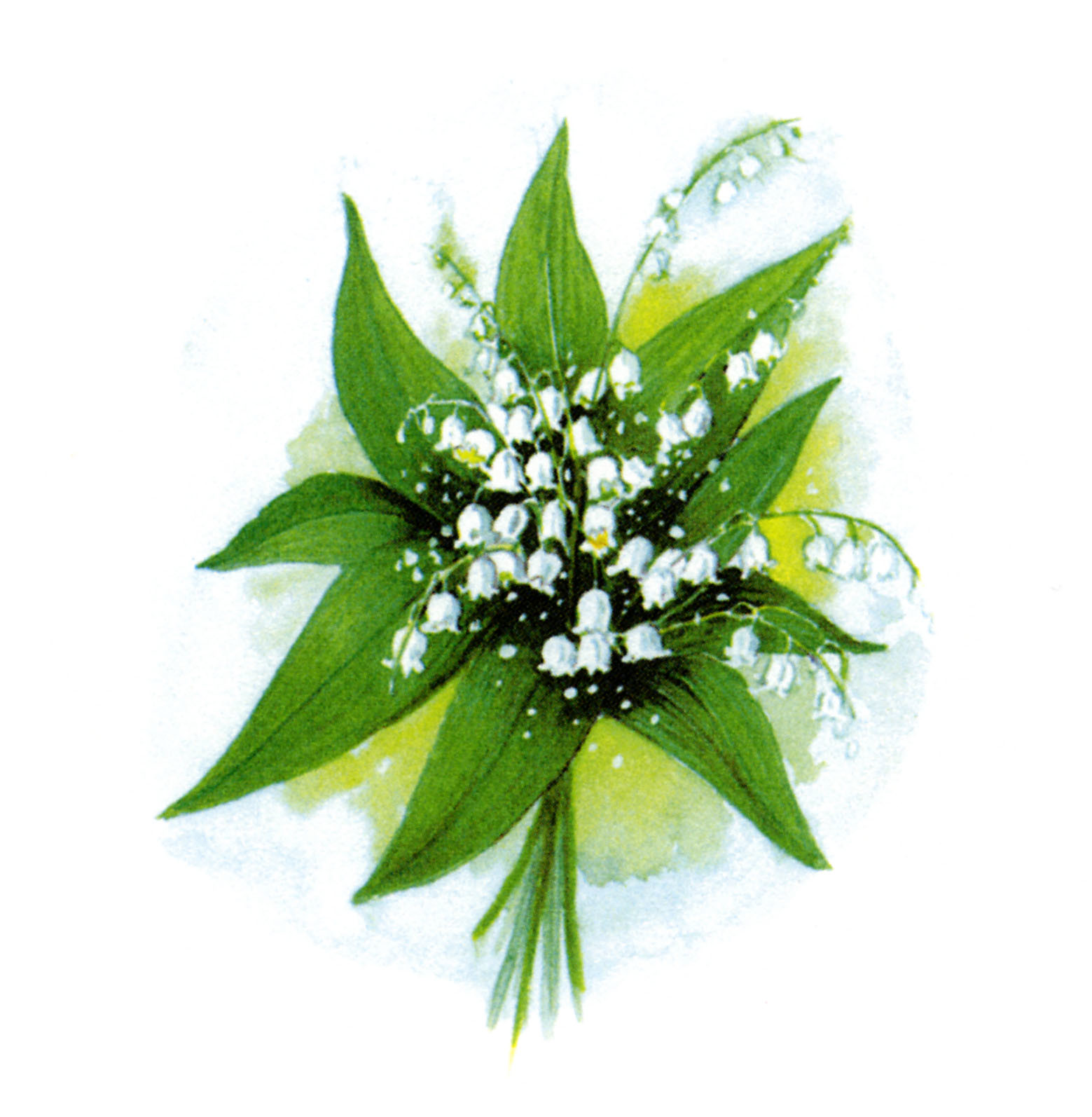The image is a detailed painting of a bouquet of lily-of-the-valley flowers, set against a white background. The delicate, bell-shaped white flowers radiate outward from multiple long and short stems, surrounded by a lush bed of dark green, pointed leaves. These leaves emanate outward in a circular formation, accented with a greenish-yellow hue and further highlighted with subtle blue undertones. Adding to the intricate composition, some flowers feature yellow centers, and a light gray, watercolor-like effect adds depth and texture to the background. The painting remains unsigned and undated, presenting a calm and cooling aesthetic.